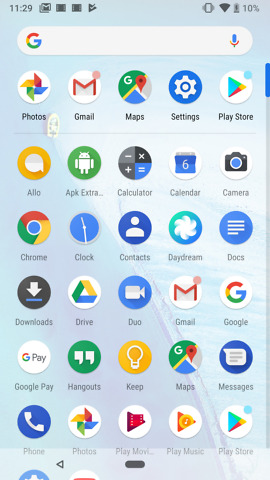Screenshot of an Android smartphone home screen featuring a standard grid layout of application icons. The icons are organized neatly in several rows and columns, offering easy access to various apps. The top row includes the "Photos" app, followed by "Gmail," "Maps," and "Settings." The second row includes the "Play Store," "Allo," and "APK Extra." Further down, you'll find utility apps such as "Calculator," "Calendar," and "Camera," as well as browsing tools like "Chrome." Essential apps like "Clock," "Contacts," "Daydream," and "Docs" are also visible. The "Downloads" folder, "Drive" for cloud storage, and the video calling app "Duo" are present. Oddly, "Gmail" appears again, followed by "Google," "Google Pay," "Hangouts," "Keep," "Maps," "Messages," "Phone," "Photos," "Play Movies," "Play Music," and "Play Store" once more. Each app is depicted with its distinct icon, making for a visually cohesive and functional home screen.